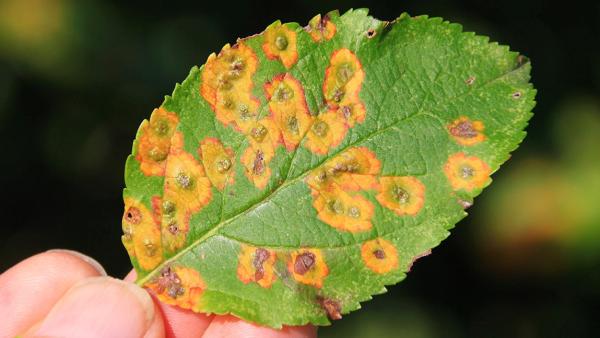A close-up image reveals a vibrant green leaf with distinct signs of disease. The oval-shaped leaf, held delicately by the fingers of a Caucasian individual on the lower left side of the image, features a prominent central vein and a pointed tip. The edges of the leaf are adorned with small, sharp spikes. The most striking feature of the leaf is the numerous yellow spots scattered primarily on its left side, each surrounded by a reddish-brown border and a greenish-brown bump at the center, some of which appear crusty and moldy. These spots merge in some areas while remaining isolated in others, further emphasizing the leaf's unhealthy state. The background is artistically blurred with a strong bokeh effect, drawing full attention to the detailed textures and colors of the diseased leaf.